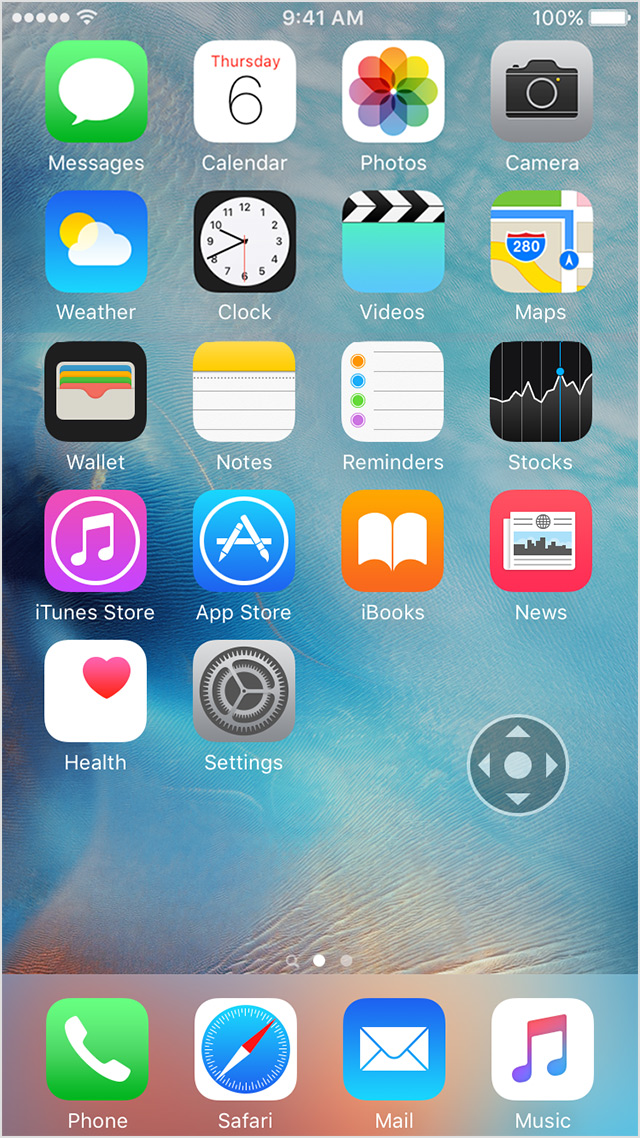The image depicts a cell phone screen displaying the home interface. At the top, the status bar shows WiFi and cellular signal strength, the time as 9:41 AM, and a fully charged battery at 100%. The screen is populated with a variety of app icons including Messages, Calendar, Photos, Camera, Weather, Clock, Videos, Maps, Wallet, Notes, Reminders, Stocks, iTunes Store, App Store, Books, News, Health, and Settings.

At the bottom of the screen, there are four persistent dock icons for Phone, Safari, Mail, and Music. Additionally, there is an icon with a distinctive design: a circle with an inner circle and triangles pointing in various directions, likely for navigation purposes.

The background wallpaper transitions from a turquoise color at the top to a light tan color at the bottom, though the abstract colors and numerous icons overlaid make it difficult to discern any specific image. The color palette includes shades of green, blue, yellow, orange, red, purple, black, gray, white, and pink, which may be part of the abstract nature of the wallpaper design.